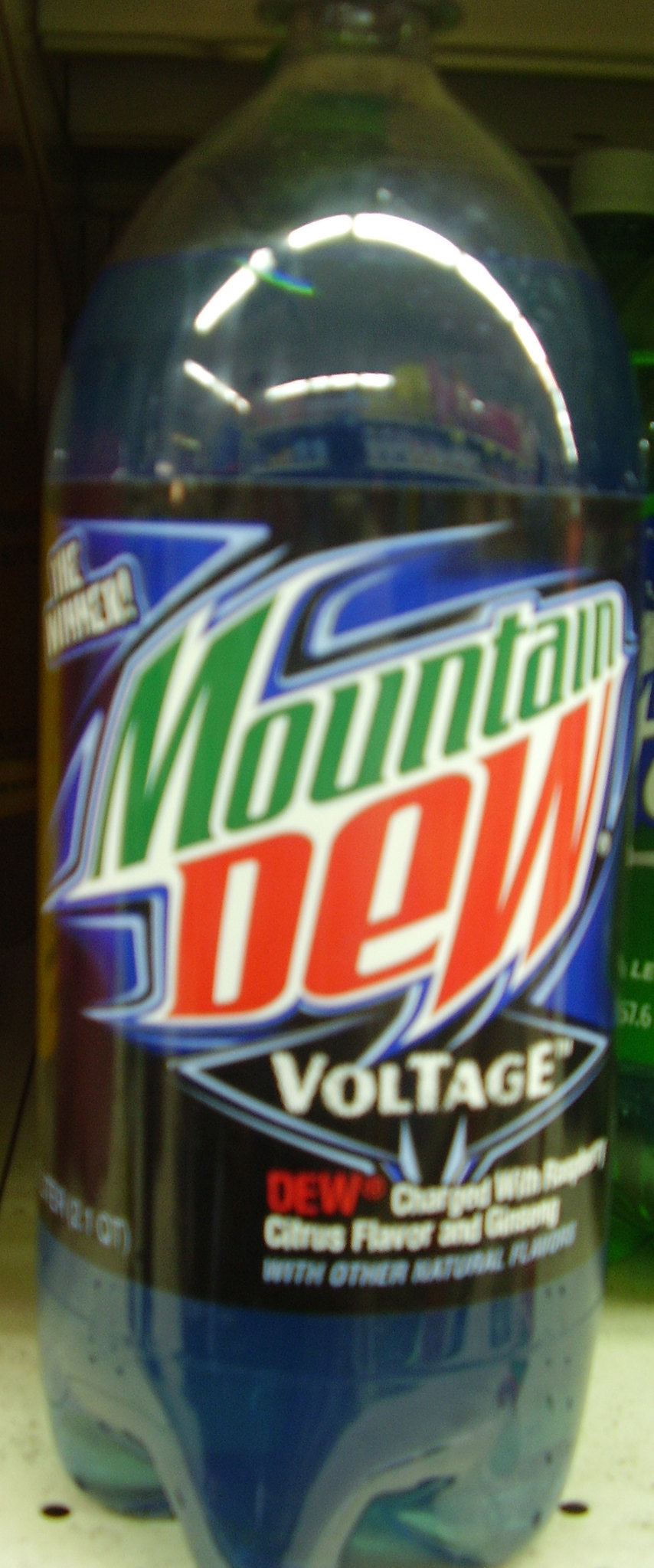This photograph captures a 2-liter bottle of Mountain Dew Voltage prominently placed against what appears to be the inside of a cabinet or possibly a shelf in a store. The bottle, made of transparent plastic, contains a blue, slightly green liquid and is around two-thirds full. The label is black and wraps around the center of the bottle. The words "Mountain Dew" are written diagonally, with "Mountain" in green and "Dew" in red. Below this, a diamond shape features the word "Voltage" in white print. The label also includes the text, "Dew charged with raspberry citrus flavor and other natural flavors," albeit slightly blurry and difficult to read clearly in the photograph. The background subtly reveals the tops of other bottles, adding context to the setting. The image also captures reflections of fluorescent room lights, curving across the surface of the bottle.